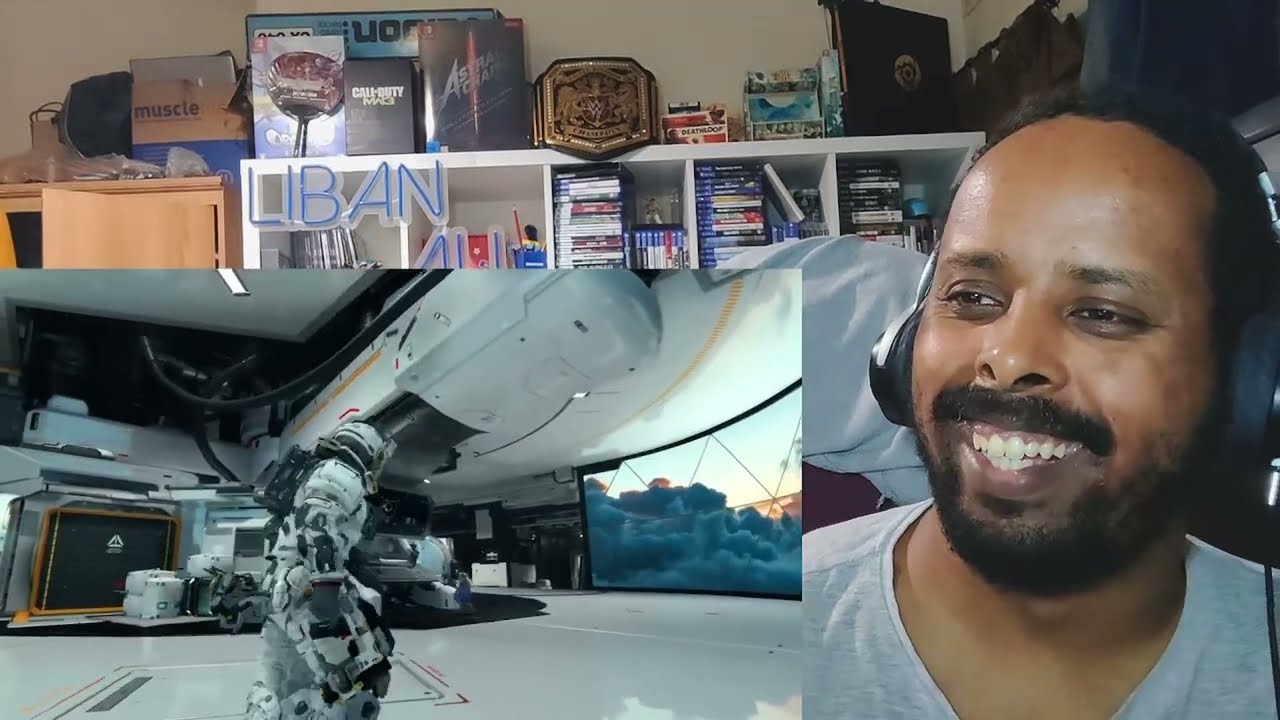The image features a man with a dark skin tone, short black hair, a mustache, and a small beard, smiling while looking sideways. He is wearing a white t-shirt and headphones, and is positioned on the right side of the screen. Behind him is a white shelf cluttered with numerous items including video games, books, possibly a wrestling belt, and movie-related paraphernalia, creating a busy backdrop. On the left side of the image is a separate screen depicting a scene that appears to be from a video game or movie, showcasing a white, futuristic environment. In this scene, a character resembling a cyborg or an astronaut stands in a lab-like or spaceship setting with smooth white surfaces and gray lines. There's also a screen on the right side within this scene, showing clouds, suggesting a window view, and adding to the futuristic vibe. This dual imagery captures both the man's reaction and the detailed, sci-fi environment of the secondary screen.